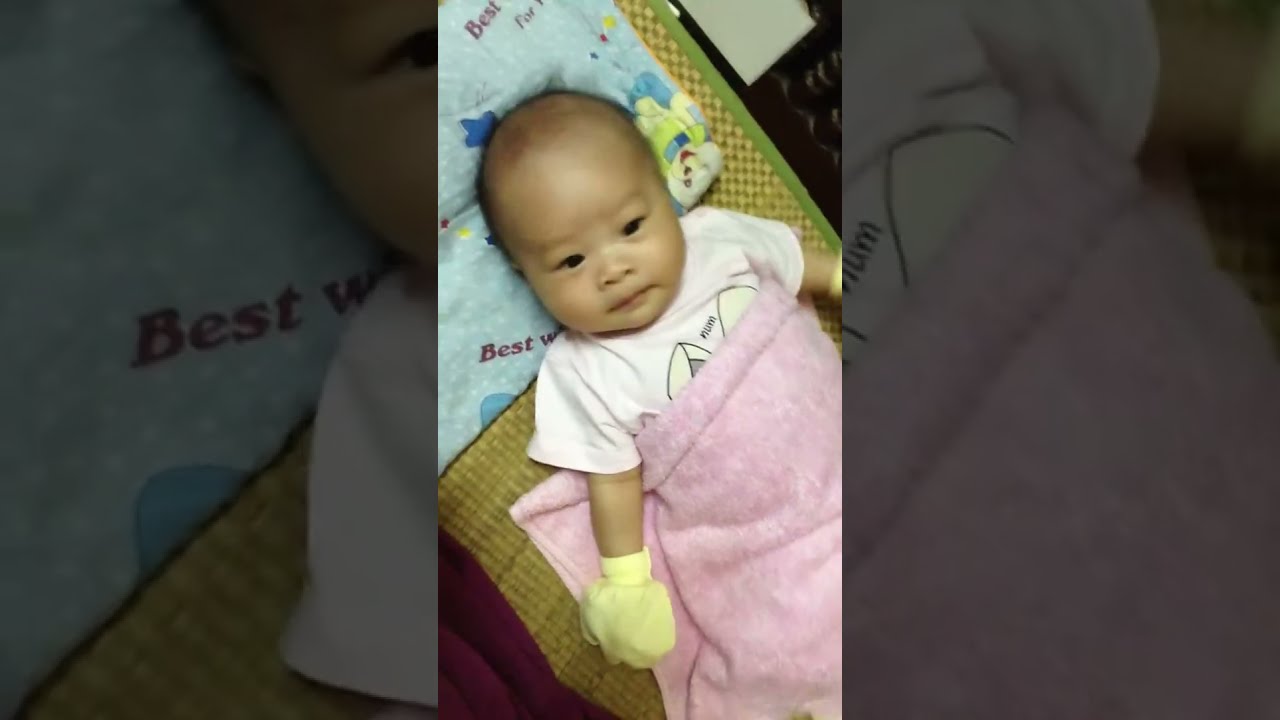This detailed image showcases a baby resting comfortably indoors, possibly in a nursery or baby's room. The photograph is divided into three panels: the left and right panels feature a black background, while the larger central panel contains the baby. The baby's head is positioned in the top-left section of the central panel, and the body extends diagonally down and to the right. The baby lies on a yellow, mesh-like pad with a green border, with a folded blanket—potentially featuring dog graphics—under its head. 

The baby is dressed in a short-sleeved white onesie and yellow mittens, likely to prevent scratching. A pink blanket covers the baby from the chest down, with the words "best wishes" partially visible, and there is a blue blanket with white specks under their head. The baby's surroundings include a woven reed mat that adds texture to the scene. Overall, the vibrant colors in the image—blue, white, pink, yellow, green, brown, black, red—contrast beautifully against the backdrop, highlighting the serene and tender moment captured from an overhead perspective. The baby's visible hair suggests they are at an early stage of growth, adding to the tender feel of the image.